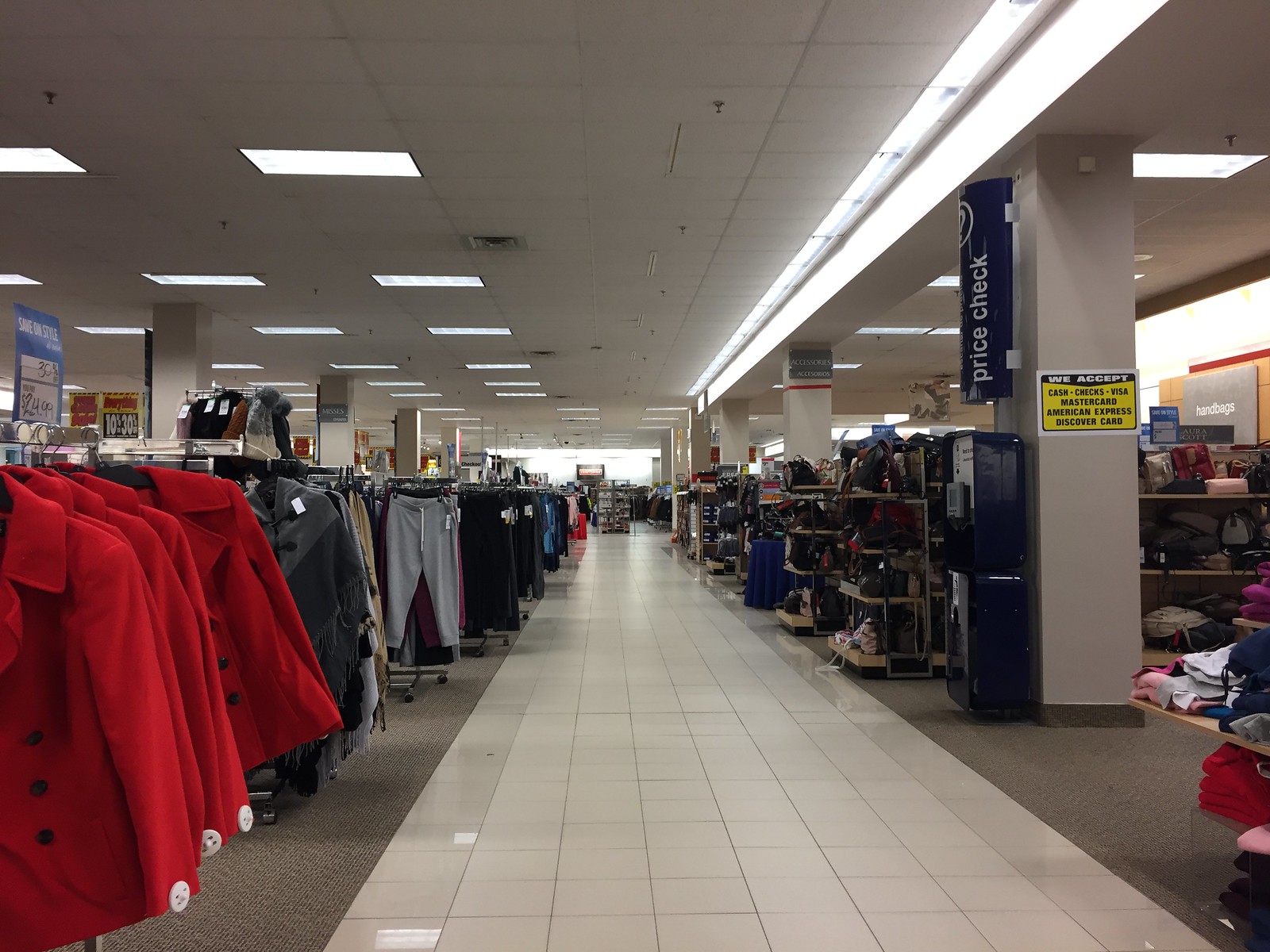This color photograph captures the bustling interior of a large department store, illuminated by a grid of fluorescent lights set into a drop-tile ceiling. The spacious store features wide white-tiled aisles and multiple structural columns. On the right-hand side of the image, the nearest column displays a sign indicating payment methods accepted at the store, which include cash, checks, Visa, MasterCard, American Express, and Discover Card. Below this sign, a blue and white "Price Check" sign is mounted above a price-check machine facing the aisle.

In the foreground to the right, there are displays of clothing, shoes, and handbags clustered together. The left-hand side of the aisle showcases a vibrant collection of red coats and a variety of pants. Sale signs are prominently placed, drawing attention to discounted items. The merchandise is arranged on a rather mundane gray carpet. The overall scene is well-lit, suggesting that it is daytime, and the vastness of the store is evident, hinting at an extensive array of products available for shoppers.